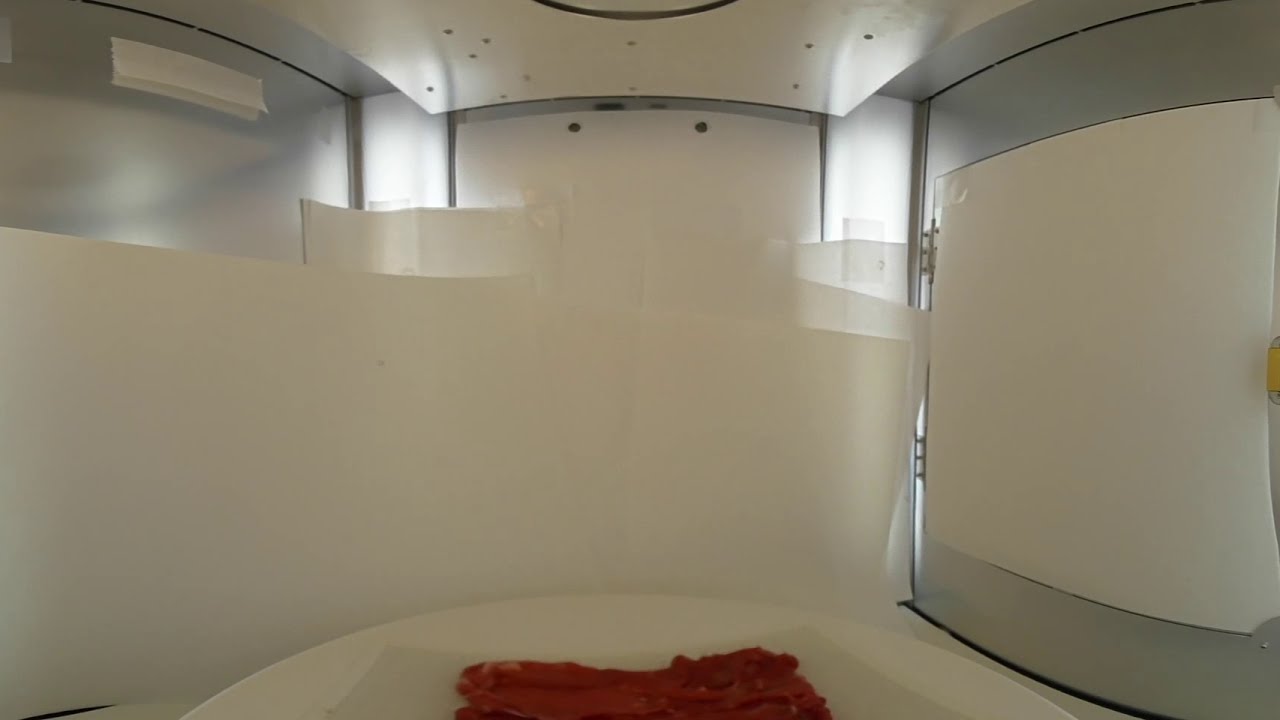The image captures a slightly distorted, fisheye perspective of what seems to be an interior, likely of a microwave or an oven. The dominant color theme is white with subtle gray trimmings. The backdrop curves gently, reminiscent of the Guggenheim Museum's architectural style, creating an illusion of spaciousness and softness in the overall setting. Central to the image's lower portion, occupying less than 5% of the frame, lies a red object—possibly a pillow, piece of clothing, or even a food item such as bacon or pizza—placed on a white surface. The scene is bathed in unusual lighting, which varies from typical kitchen microwaves, lending an enigmatic quality to the space. To the right, a panel decorated with a white rectangle bordered by a light gray frame repeats the theme, enhancing the room’s minimalist aesthetic. The perspective hints that the photograph might have been taken with a smartphone or tablet, capturing the peculiar angles and lighting that add to the overall mystique of the image.